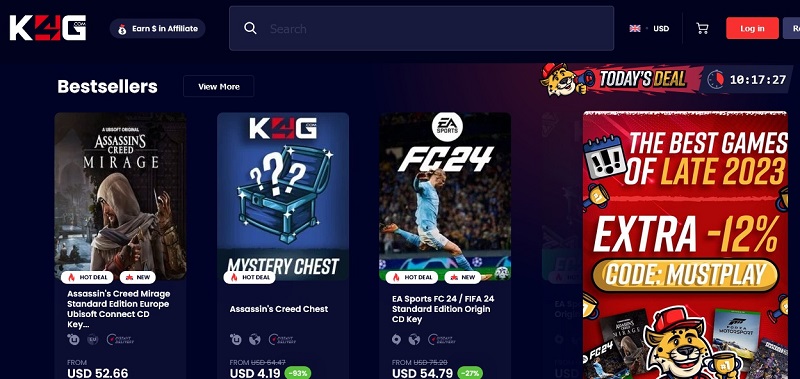This image showcases the homepage of a gaming platform website, K4G.com. The top left corner features the K4G logo, with white 'K' and 'G' letters and the number '4' inside a red box. Adjacent to the logo are buttons labeled "Earn Money" and "Affiliate." A search bar is positioned to the right, against a dark background which appears either black or very dark blue. Further right, there are options to log in and access a shopping cart. 

Directly below this header, a section titled "Today's Deals" is prominently displayed, accompanied by a clock icon, suggesting that the deals are time-sensitive. Above the K4G logo, there is a "Best Sellers" section with a "View More" button for additional items. 

The primary content features various game offerings, including an artwork for "Assassin’s Creed Mirage" with the description "Crescent Seed Mirage Standard Edition Europe Ubisoft Connect CD Key." To the right, there are promotional boxes for the "K4G Mystery Chest" and "Assassin’s Creed Chest." Lastly, there is another game feature for "EA Sports FC24," also referred to as "FIFA 24," available as the "Standard Edition Origin CD Key."